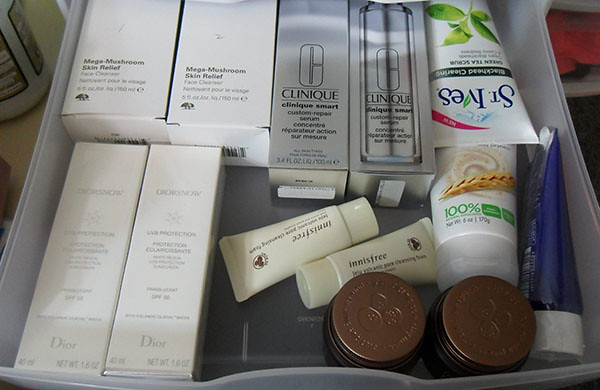In this image, a clear pulled-out plastic drawer showcases a variety of skincare products meticulously organized. Starting from the upper left-hand corner, there are two white boxes labeled "Mega-Mushroom Skin Relief Face Cleanser" in green print. Positioned below these, there are two white Dior boxes, each stating "Net Weight 1.6 oz, SPF 50, UVB Protection," although the text appears somewhat faded and challenging to read. Next to them are two silver-colored boxes branded with "Clinique Smart Custom-Repair Serum." Additionally, there is a white bottle adorned with a green leaf pattern that reads "St. Ives Green Tea Scrub Blackhead Clearing." Further to the right, two circular jar containers with bronze-colored lids stand out. Finally, a white and blue tube, the text on which is not visible, sits on the extreme right side of the drawer.